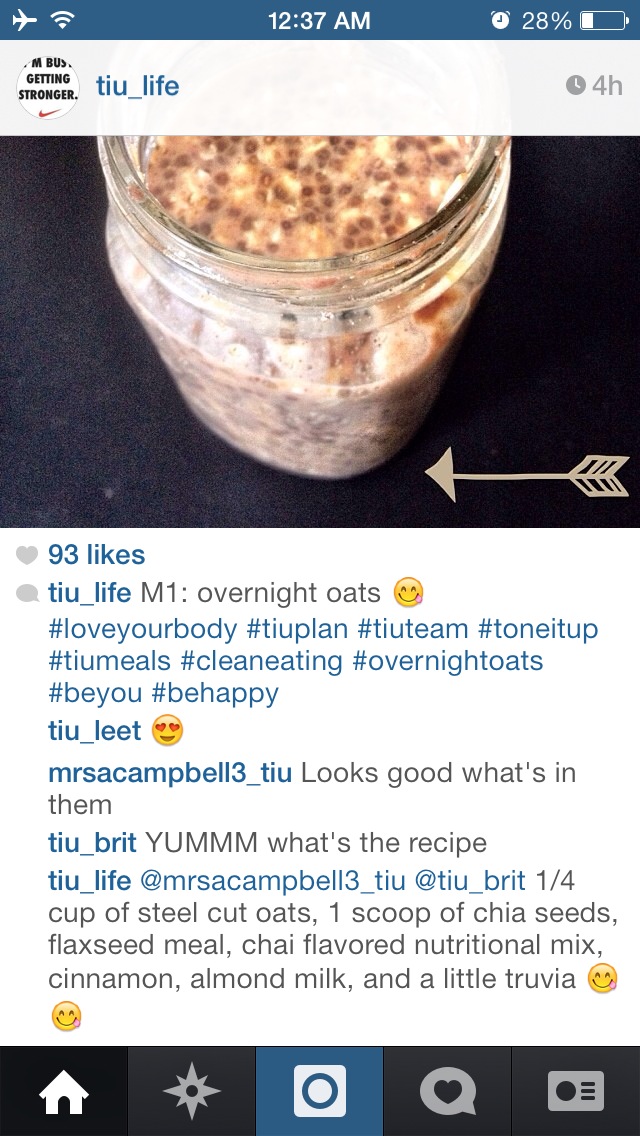This screenshot from a phone, taken at 12:37 a.m. with the phone in airplane mode and a battery charge of 28%, captures a social media post by the user T_I_U_L_I_F_E. The post, created about four hours ago, features a glass jar filled with a mixture identified as overnight oats. This nutritious meal includes steel cut oats, a scoop of chia seeds, flaxseed meal, chai flavored nutritional mix, cinnamon, almond, and a touch of Truvia, all detailed in the recipe shared in the post. The post, which garnered 93 likes, is heavily hashtagged with terms like love your body, TU plan, TU team, tone it up, TU meals, clean eating, overnight oats, be you, and be happy. The screenshot also shows a series of icons at the bottom, representing different interaction options available within the app.